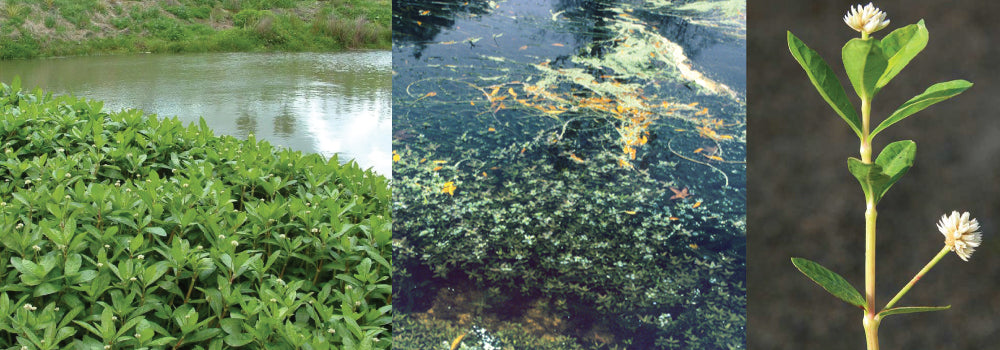A three-panel nature photograph captures different scenes of a lake or swamp area. The far left image showcases a swampy lakeshore with green plants at the bottom, murky brownish-gray water in the middle, and reflections of trees, clouds, and sky above a small grassy bank at the top. The middle panel presents a more polluted part of the lake where a whitish-orange algae bloom or some contaminant floats on the surface. Beneath this, greenish plants with small white flowers are visible, indicating submerged vegetation. The rightmost image is a close-up shot of a single plant with green leaves and spiky white flower buds. This plant might be the same as those appearing in the far left image, providing a detailed view of the floral elements in the scene.